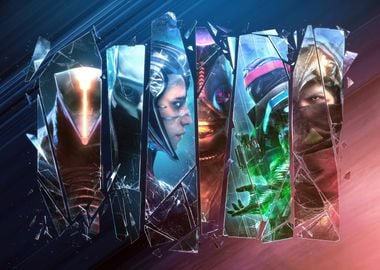This image appears to be a digital poster or box art for a video game, characterized by a striking and vibrant color scheme. The background is split into shades of pink, blue, and red, creating a dynamic and visually engaging setting. Across the front of the poster, there are shards of shattered glass, each containing a different character from the game. These fragments create a collage effect, emphasizing the diversity of characters.

In the center shard is a man wearing a helmet, suggesting a lead role. Another shard features a woman, distinguished by her visible hair and eyes. Additionally, there is an intriguing character on the rightmost shard with their face obscured by cloth, revealing only their eyes, adding an air of mystery. Some shards also depict alien-like figures, hinting at the game's potential sci-fi or fantasy elements.

The overall color palette is dominated by blue, with significant accents of red, dark blue, green, and pink, giving each shard and character a unique visual theme while maintaining cohesion across the poster. This composition effectively captures the essence of the game, poised to attract viewers with its vivid imagery and intriguing character lineup.